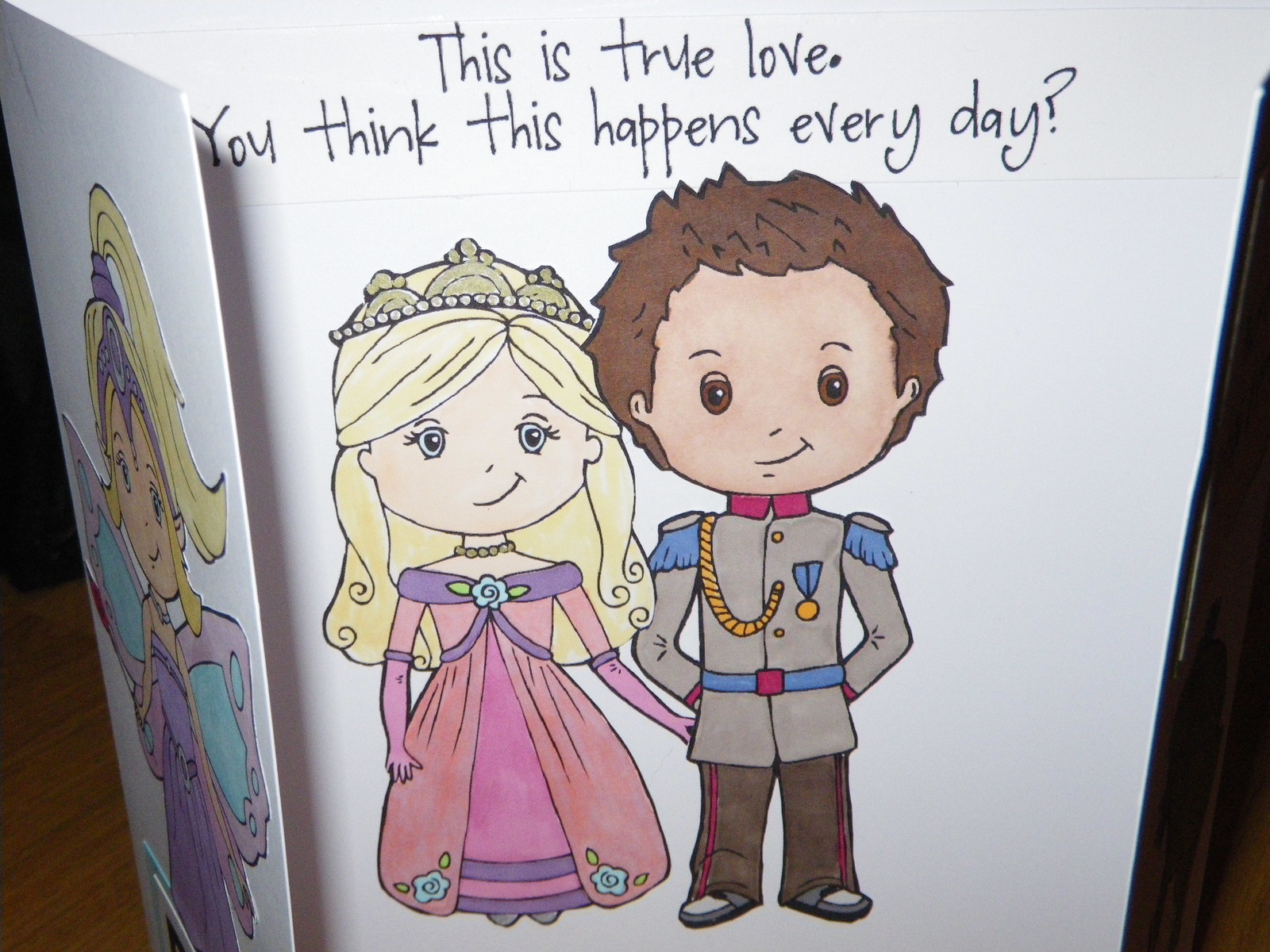This image depicts an opened, white paper card, displaying both the inside and a glimpse of the front cover. The card features charming, colorful illustrations of a prince and a princess. The princess, with her long, curly blonde hair adorned with a crown, is dressed in a pink and purple gown. Her enchanting style is complemented by butterfly wings painted in light purple and teal. The prince beside her has short brown hair and is depicted in a gray, military-style jacket adorned with medals and dark-colored pants. They are shown holding hands, both smiling warmly. The text at the top of the card reads, "This is true love. Do you think this happens every day?" This whimsical design, reminiscent of fairytale characters like Cinderella, creates a magical and romantic atmosphere.